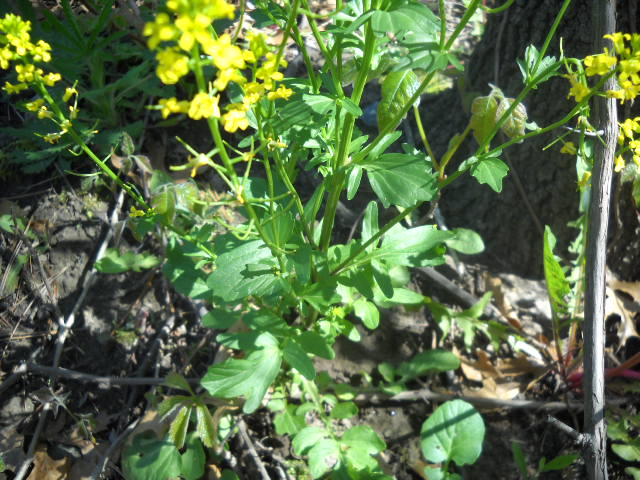This close-up photograph captures an outdoor scene bathed in natural light, with some areas in shadow. The focus is on a dense patch of green foliage featuring long stems with leaves interspersed with vibrant yellow flowers. The scene is set on a dirt ground littered with numerous crisscrossed twigs. On the right side, there is an upward growth of twigs that resemble vines. A sloping tree trunk is visible at the base, partially cut off by the frame. Surrounding the main plant in the middle, which has green stems and yellow flowers, are more plants of a similar nature with green branches and leaves. Additionally, remnants of a small wooden fence are visible, including pieces of wood on the ground and a wooden pole extending nearly to the top of the image. The background features more of this lush foliage and a hint of a path.